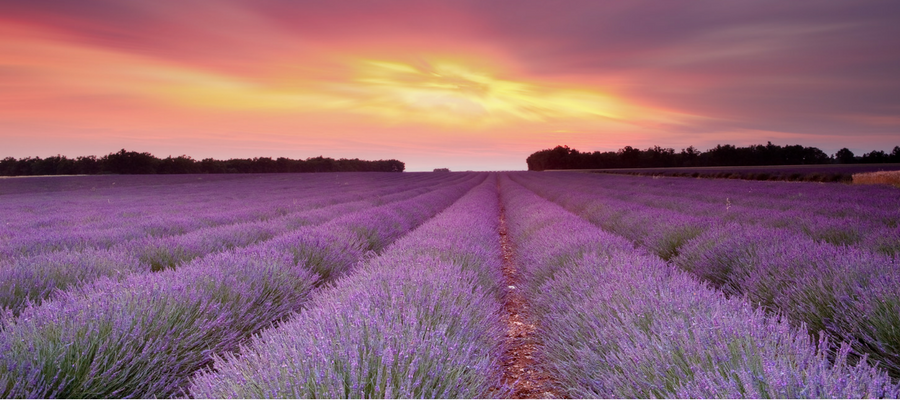A breathtaking lavender farm extends into the distance, with meticulously arranged rows of vibrant purple flowers. The green foliage beneath the lavender adds a rich contrast, and patches of dry, brown soil delineate each row. In the distant horizon, a stunning sky transitions from a pinkish-yellow near the center to deep orange and dark purple overhead. The golden hues again blend into orange closer to the horizon. Lining the far edges of the field, a scattering of trees can be seen predominantly on the right and left sides, framing this picturesque landscape.